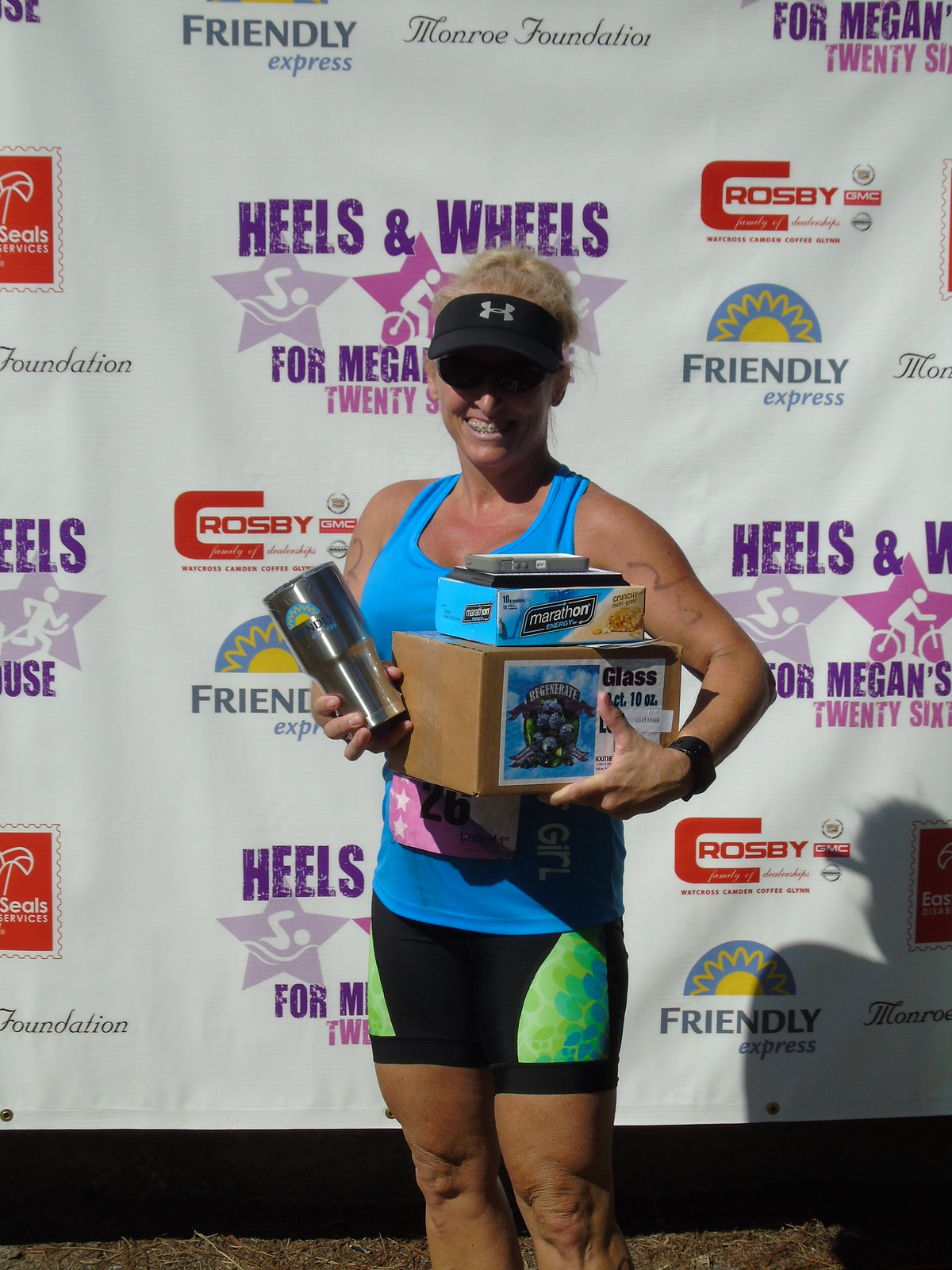In the image, a woman is standing in front of a white backdrop covered with numerous logos, including "Heels and Wheels," "Crosby," "GMC," "Friendly Express," "Monroe Foundation," and "For Megan 26," though some text is cut off. The wall is adorned with various logos and triathlon symbols. The woman, whose face is partially obscured by a shadow cast from a black visor with the Under Armour logo, has blonde hair peeking out. She is dressed in a blue tank top and black biking shorts with green insets, which might appear red with green pockets in some areas. She holds several items: in her left hand, a silver sports cup with a Sunshine logo and a thermal cup, while her right hand holds a cardboard box labeled "glass" alongside a picture, topped with a Marathon box that possibly has a phone or stack of cards on it. There’s also a purple tag, perhaps a name tag, under her chest, largely hidden by the box. The overall setting and her athletic attire suggest she may have just won a sporting event.